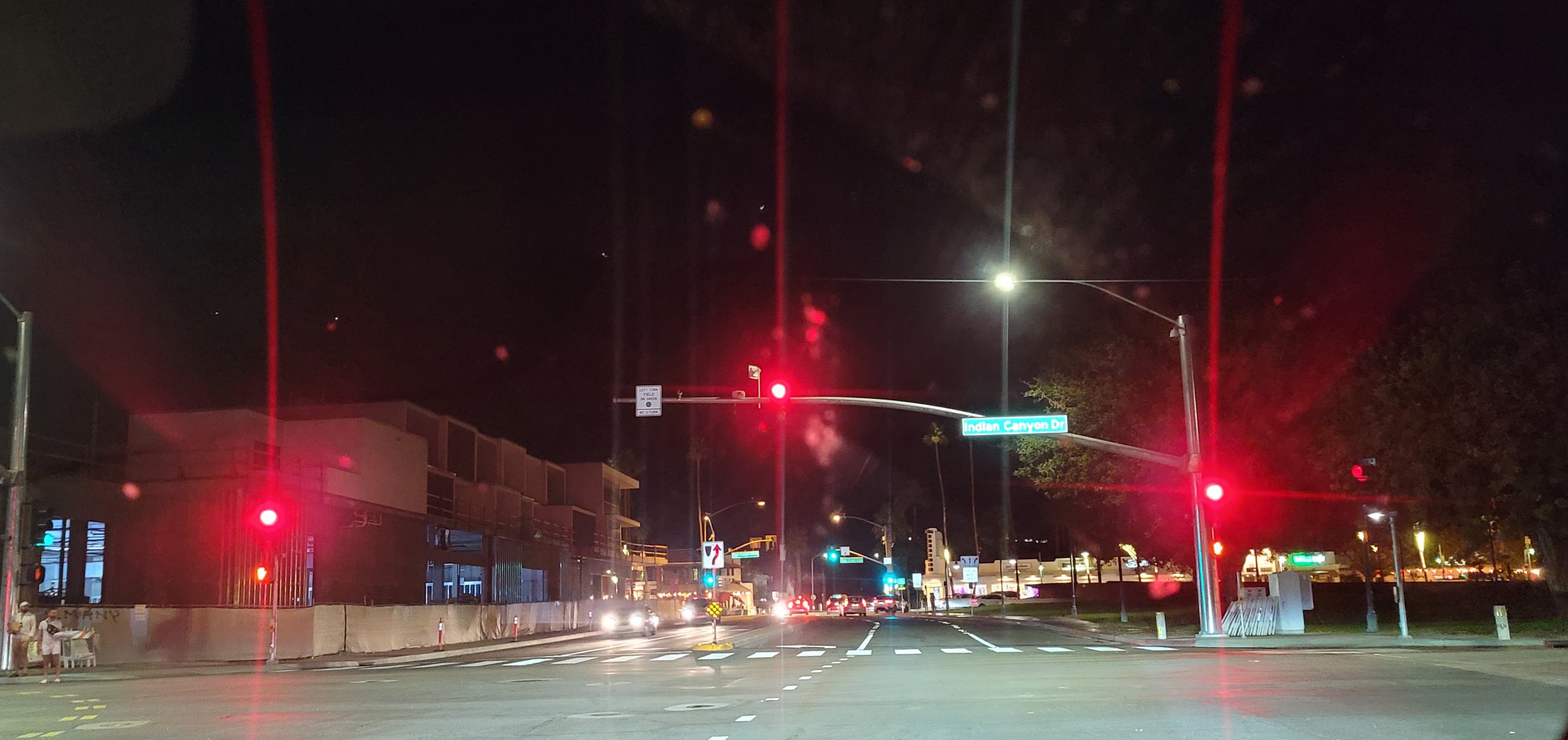A wide-angle night shot captures a quiet intersection from inside a car, evident from the dirt-speckled windscreen at the top center of the image. The scene is dominated by the illuminated streetlights, casting a stark contrast against the dark surroundings. The image's dimensions are roughly 2.5 times wider than its height, offering a panoramic view.

In the foreground, an expansive intersection can be seen devoid of immediate traffic, indicating the car is likely in the front row. On the far side of the street, a couple of vehicles approach, their headlights cutting through the night. A significant vertical streetlight stands on the roadside, its single lamp brightly shining. Beneath it, a green street sign is partially visible, though the text is unreadable.

Extending from the streetlight is a horizontal bar with several lights. Among them, a primary red traffic light glows intensely, accompanied by another red light on the opposite left side of the road, contributing to a star-like lens flare effect. There’s also a left-hand turn signal or perhaps a white square sign at the bar’s end. A stark white streetlamp higher in the background illuminates the intersection, casting a broad beam downwards.

Across the way, a concrete divider slices through the opposite road, marked with a downward-arced oval avoidance sign and an arrow veering right. Although distant vehicles may be receding into the dark, they remain indiscernible. To the left, a commercial building or condominium rises two or three stories high against the night sky. On the right, past the intersection, a vacant lot or park comes into view, flanked by a cement wall roughly two to three feet tall, topped with a fence, lining most of the visible street. The atmospheric shot subtly reveals the stillness of a late-night urban environment.